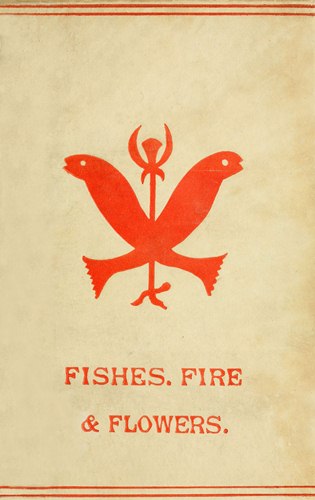This image is a vertical, rectangular poster with an aged, parchment-like background that has a worn, yellowish cream color with some brown tarnished edges, giving it an old-fashioned appearance. The poster is bordered on the top and bottom by two horizontal red lines. In the center of the poster, there is a red emblem featuring two red fish, each seen in profile, facing opposite directions and intersecting to form an X shape with their bodies. In between the intersecting fish, there is a symbol resembling a forked tool or stand with two prongs and a middle stick, possibly representing a flower. Below the emblem, the text reads in all capital letters: "FISHES, FIRE, & FLOWERS."